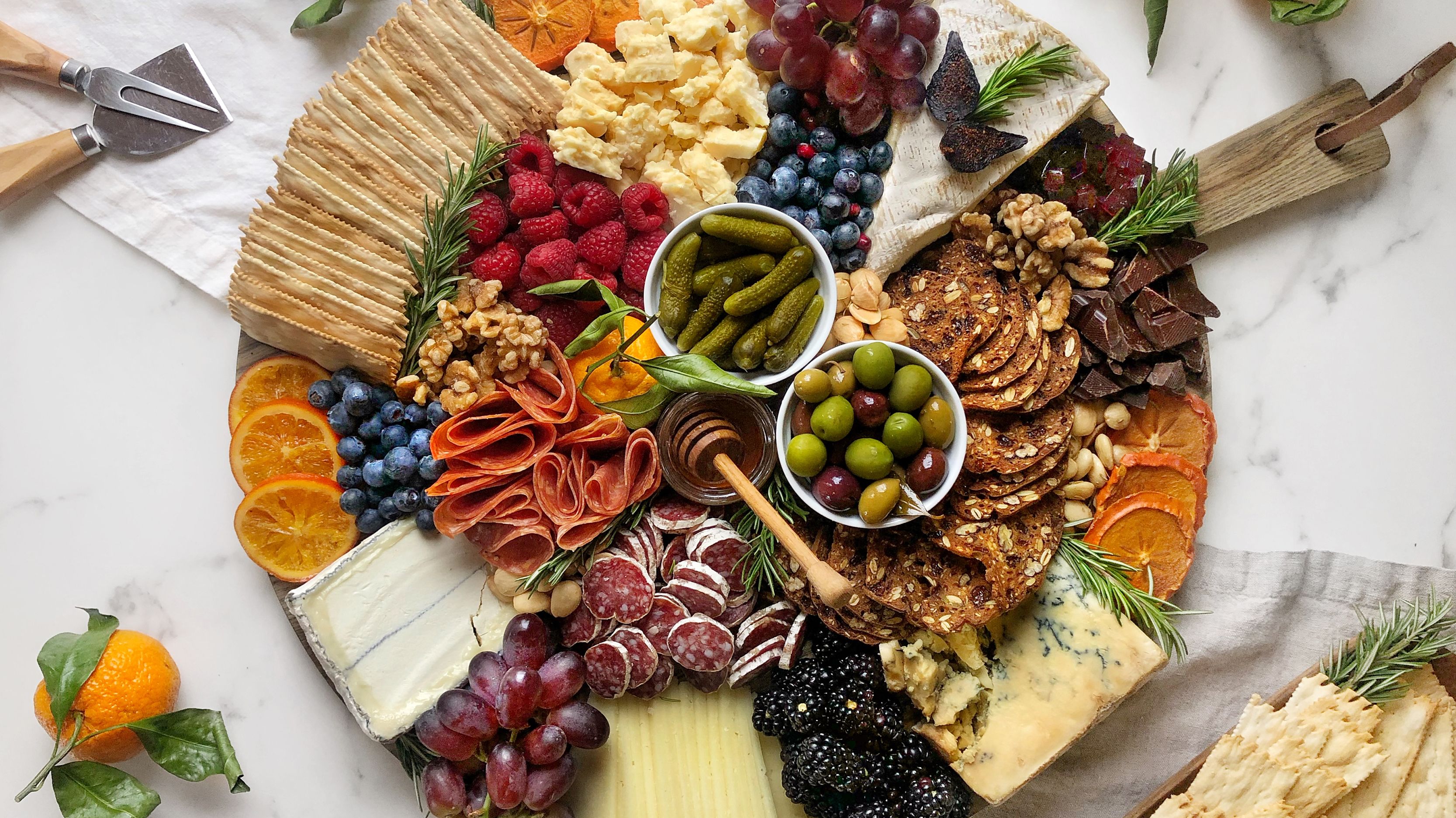The image is a stunning, overhead view of a beautifully arranged charcuterie board, placed on a marble countertop. The round wooden board, adorned with a leather-strapped handle in the upper right corner, displays a sumptuous assortment of gourmet delights. A white linen napkin rests under one side of the board, providing an elegant touch alongside a specialty cheese paddle and cheese fork in the upper left corner.

The charcuterie board is meticulously organized, beginning with fresh blackberries at five o'clock and moving counterclockwise to include blue cheese, slices of soppressata or salami, and fresh orange slices. Blanched almonds, wedges of chocolate, and sprigs of rosemary add both flavor and visual appeal. There are also walnuts, dried cranberries, and a large wedge of brie topped with a cut-open dried fig.

In the center, small bowls hold gherkins, a variety of green, yellow, and red olives, and honey with a wooden drizzle utensil. The array extends to include blueberries, red grapes, and persimmon slices. Rolled-up ham slices, a block of soft cheese, and narrow slices of salami with a whitish rind complete the assortment. Also visible are raspberries, round cheeses, and flatbreads or crackers.

An additional glimpse of a whole orange with leaves in the bottom left, more blueberries, and extra crackers on a small wooden board with a sprig of thyme in the lower right, enhances the inviting presentation of this rich and diverse charcuterie spread.